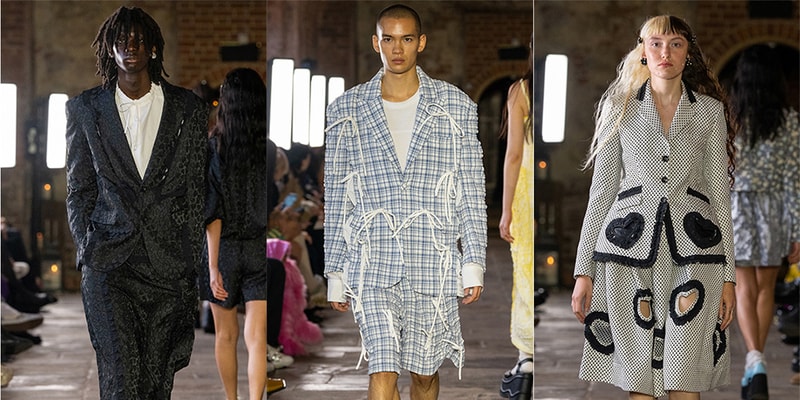This image is a composite of three rectangular photographs placed side by side, forming a wide, panoramic view. The scene is set indoors, revealing a fashion shoot or runway show within a building that has a brick background and a light gray stone floor. 

On the far left, a black male model with dreadlock-style hair is dressed in a white shirt and an oversized, shiny black suit adorned with a leopard print design. The outfit has a formal yet distinct, edgy appearance.

In the center, a male model of Asian descent with a closely shaven head dons an unconventional ensemble. He wears a white t-shirt under a distressed, oversized jacket and matching shorts with a blue and white pinstripe pattern, both uniquely embellished with white shoelace bows.

On the right, a female model of Caucasian descent features long, two-tone hair, half blonde and half brunette, styled with slight curls and short bangs. Her outfit is a light gray jacket and skirt ensemble. The jacket has prominent black polka dots and two black love hearts near the top, while the skirt displays intentional cuts and see-through holes, providing a playful yet sophisticated look.

In the background across all three photos, spectators seated on the left suggest the models are walking down a runway, further emphasizing the fashion show setting.